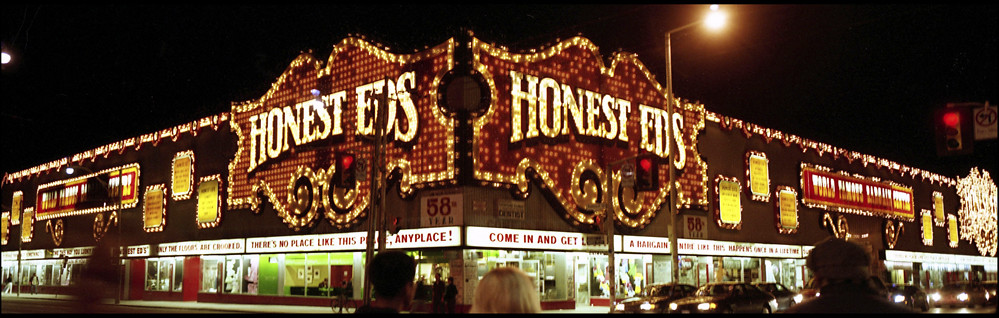The photograph captures a night scene of the street corner of a prominent two-story building named "Honest Ed's," which occupies a considerable portion of a city block. The shot places the corner of the building almost at the center of the frame. The sky is pitch black, emphasizing the illumination provided by numerous small lights adorning the building. This illumination, reminiscent of Las Vegas-style lighting, highlights the brown facade and the lighter brown signs that proclaim "Honest Ed's" on multiple sides. The building is festooned with signs touting deals and bargains, contributing to an atmosphere of a discount paradise. A sign indicating "58 years" is visible, hinting at the establishment's longstanding presence. There is a light post positioned slightly to the right of the middle of the image, flanked by moving cars on the right and the backs of people’s heads at the bottom, adding a touch of urban life to the scene.